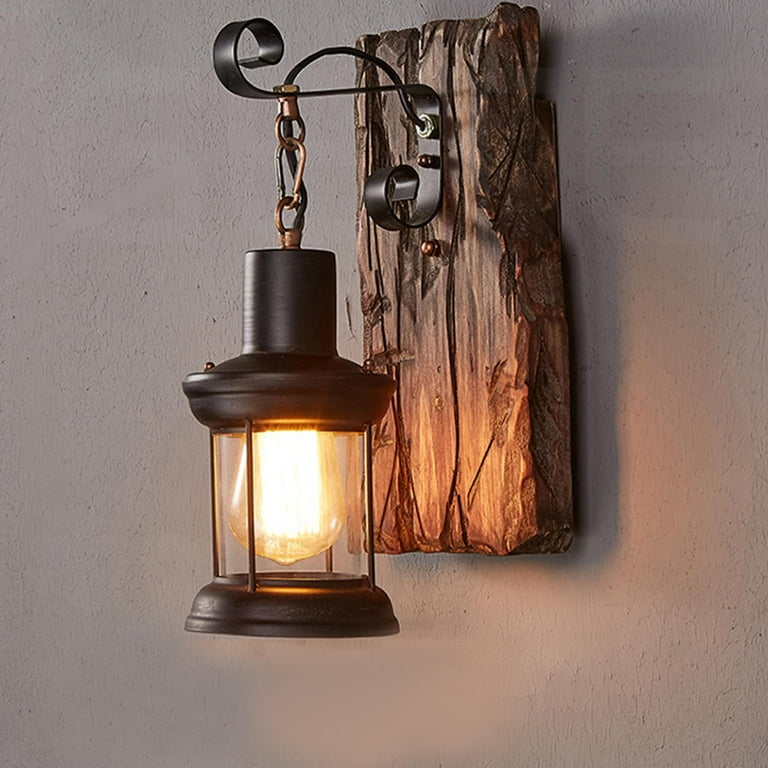This close-up photograph showcases a traditional black metal lantern-style lamp hanging from a curved, black metal bracket. The bracket is firmly attached to a rough-cut, dark brown wooden plank, which contrasts beautifully against the light gray plaster or white stone wall it is mounted on. The lantern features intricate black hardware and a cage-like structure, housing a yellow Edison-style bulb that emits a warm light. The soft glow from the bulb illuminates the base of the wooden plank and casts an orange hue onto the nearby wall, enhancing the rustic, weathered look of the wood, which bears distinct carvings and marks. The chain connecting the lantern to the metal bracket is bronze, adding a touch of vintage charm to the setup. Despite the close framing of the image, the rich textures and colors of the lantern, wood, and wall provide a vivid and detailed visual narrative.